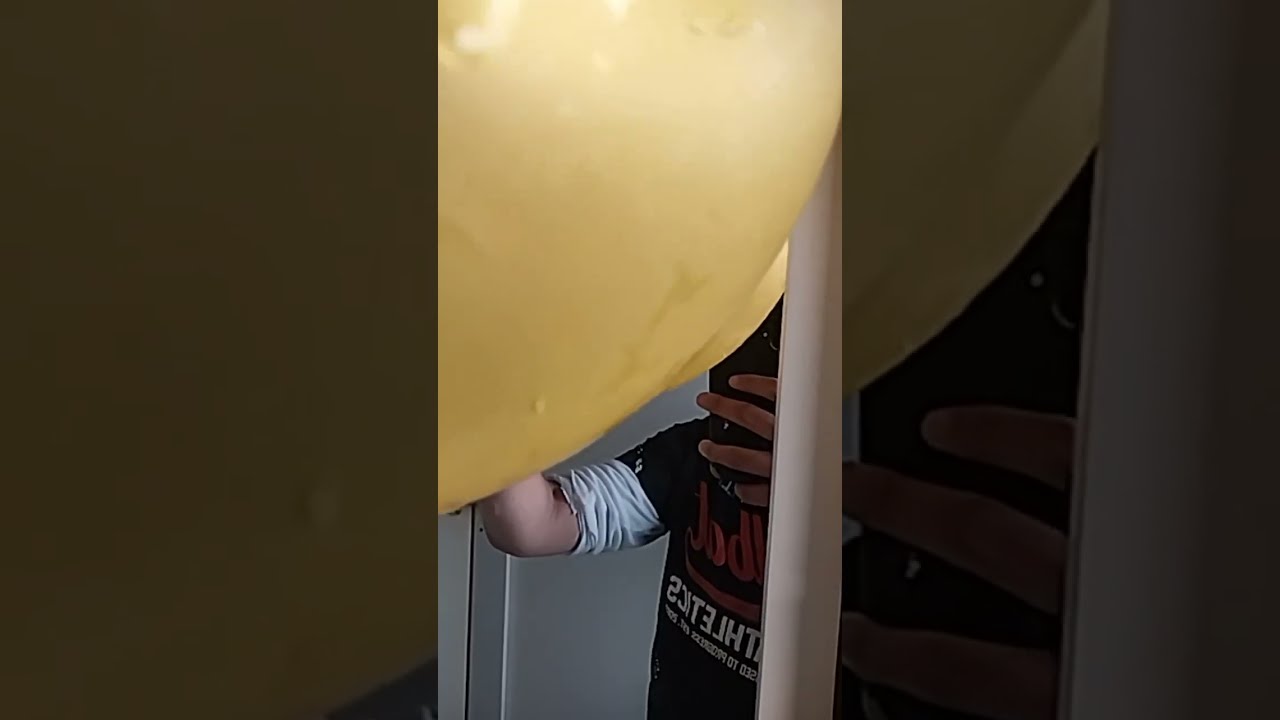The image features a visually striking composition where a vertical central strip draws most of the attention, flanked by faded and zoomed-in sections of the same image on both sides. The focal point is a person taking a mirror selfie mounted on a wall. A large, matte, yellow object—possibly a balloon or gourd—dominates the upper left portion of the image, partially obscuring the individual's face. This yellow object appears prominently in all sections of the composition, although it is fragmented and less clear on the sides.

The person in the photo is a Caucasian male wearing a layered outfit: a black short-sleeve shirt over a white long-sleeve one, with the sleeves rolled up to the elbows. He holds a phone with one hand, capturing the selfie, while his right hand is raised mid-frame. The text on his black shirt, colored in orange and white, appears reversed due to the mirror reflection. He stands in front of a white wall, framed by the large yellow object, creating a curious and somewhat ambiguous scene.